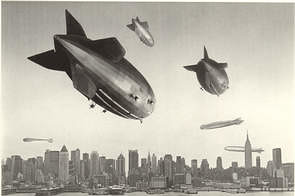The image is a small, black and white drawing that appears to have been sketched in pencil, with a muted filter overlaying the scene. It depicts a city skyline reminiscent of New York City, with several tall buildings including what looks like the Empire State Building on the right-hand side. The skyline is dotted with an array of blimp-like objects, some of which could be interpreted as wartime blimps or even missiles. 

In the foreground, there are larger blimps, one prominently close and headed toward the viewer, and two more situated above it. Further in the distance, a series of these objects can be seen moving from the right side of the image towards the left, skimming just above the tops of the buildings. One of these is positioned so low that it is below the peak of the Empire State Building. The sky transitions from a grayish hue at the top to a brighter tone towards the bottom, enhancing the surreal nature of the scene. Water can be discerned towards the bottom edge of the image, suggesting the city might be situated on a waterfront.